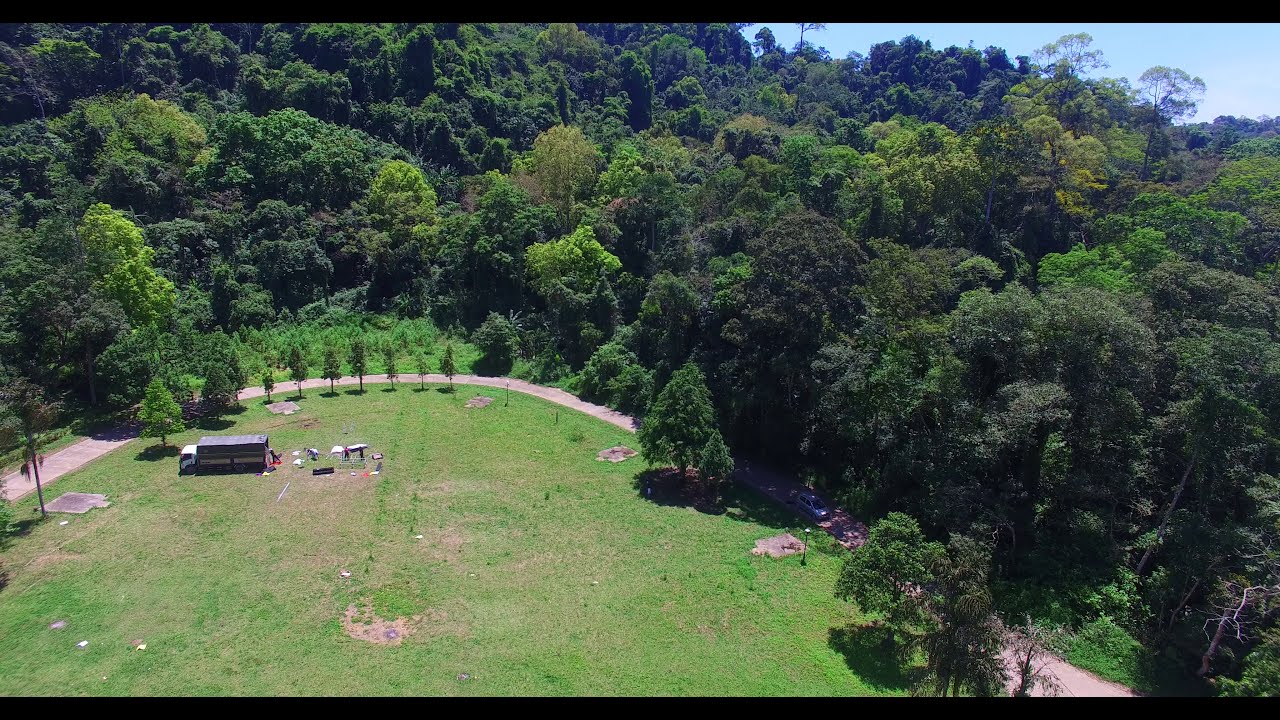A drone-captured photo, taken around 50 feet above ground, showcases a vibrant landscape composed of a lush forest and a grassy field during daytime. The forest, featuring a diverse palette of tree colors from dark green to light emerald to yellow-green, stretches upwards on a hill to the left while remaining level on the right side of the image. A road, resembling a half-oval, extends from the bottom right to the bottom left of the photo, with trees bordering it except for two located on the inside curve. At the lower edge of the image, a grassy field hosts a large, commercial gray truck with an open bed, next to which two people are standing. Picnic tables are visible near them. Additionally, the upper right corner reveals a patch of blue sky, framed by a thin black border at the top and bottom of the image.